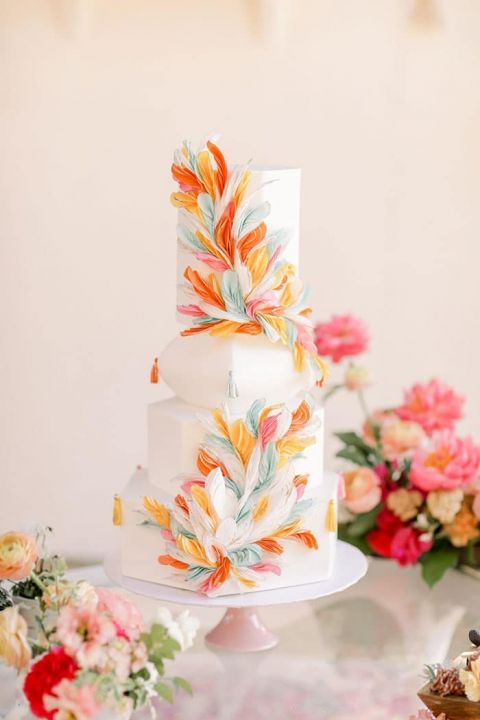This photograph features an exquisitely designed, multi-layered cake set on a glass-top table. The cake stands prominently at the center of the image, with a pink ombre background that gradually transitions from the top to the bottom. This five-tiered cake, while not exceptionally tall, boasts varied shapes in its layers, including hexagons, octagons, and a pillowy form, all enveloped in white icing. The cake is adorned with striking floral sprays made from icing in shades of white, orange, red-orange, and pale green, giving it a tropical yet delicate appearance. These flowers, possibly resembling daffodils, are intricately designed, with some appearing on the top and bottom tiers. Each layer is further embellished with small tassel-like details. Surrounding the cake stand on the tabletop are lush bouquets of flowers, featuring hues of pink, cream, red, and white roses alongside green foliage. To the right of the cake, there's a bouquet of dark pink flowers, while the left corner displays a bouquet of light pink, red, and peach flowers. A partially visible bowl with an unknown substance is situated at the bottom right of the scene, enhancing the overall elegance and intricacy of the display.